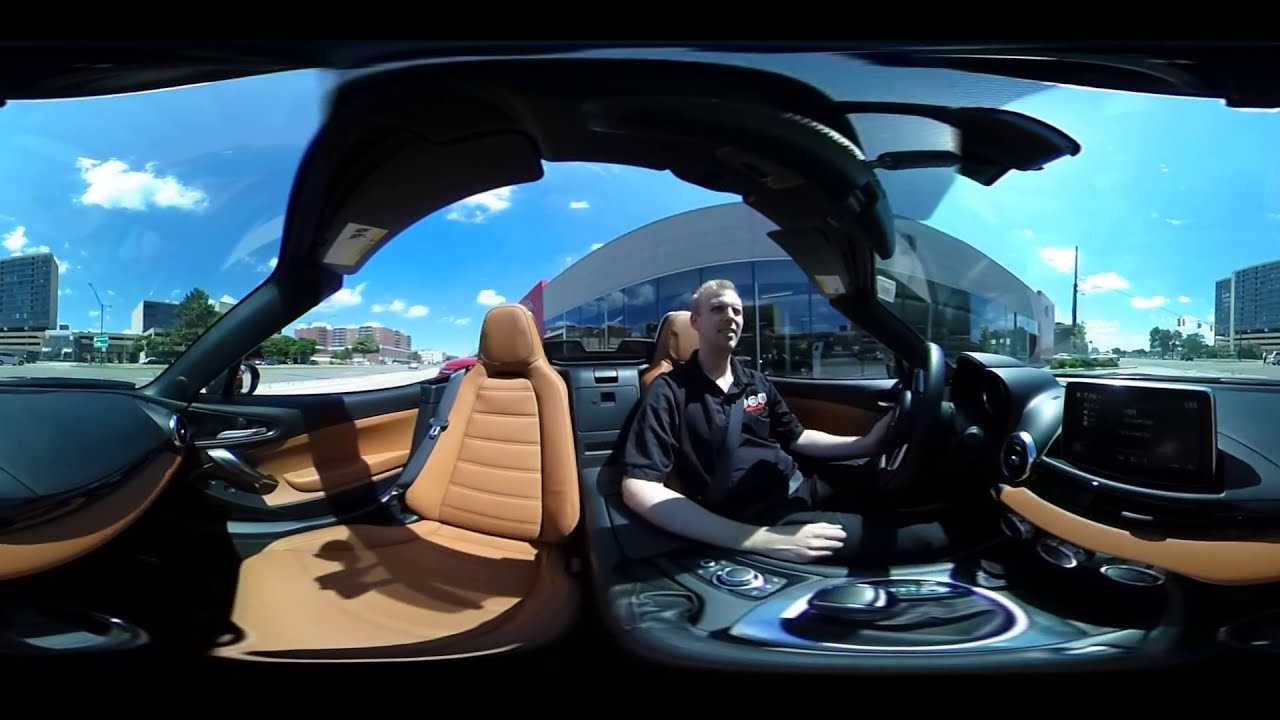The image depicts a young Caucasian man with short blonde hair, wearing a black short-sleeve shirt featuring a logo, seated in the driver's seat of a car. His hand is on the steering wheel, and he has a smile on his face. The car's interior predominantly consists of black and tan leather, with a touch screen on the dashboard. The man is centrally positioned in the frame, with some noticeable warping likely due to a virtual reality lens effect, which distorts the car's passenger seat and top slightly. Outside the car, a bright midday sky filled with scattered clouds serves as the backdrop, alongside several buildings and a road with other vehicles, suggesting a location near a dealership, perhaps post-purchase. The image is vibrant with colors including black, blue, white, gray, tan, silver, red, and green, adding to the detailed outdoor scene.